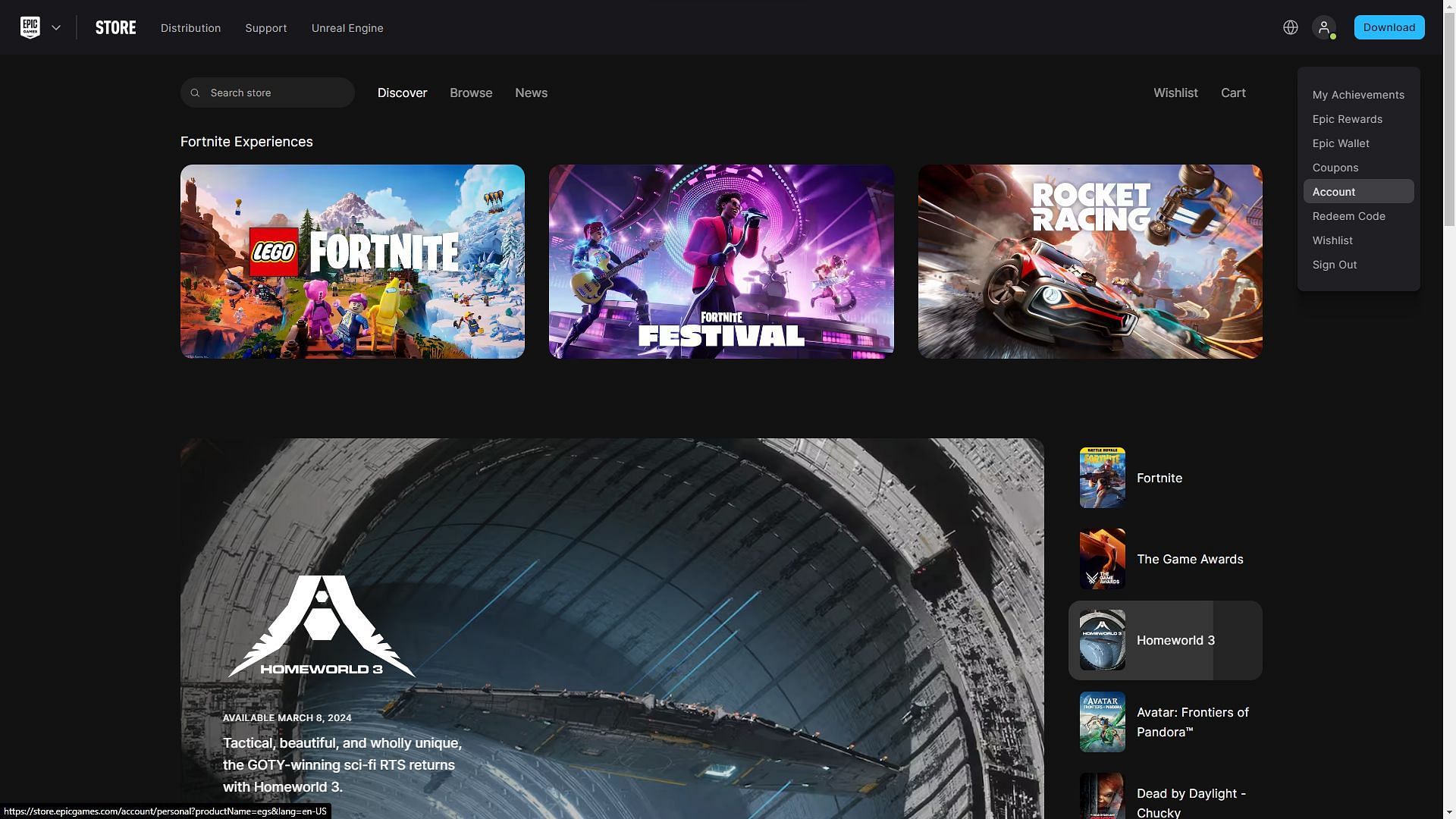Here's a detailed and cleaned-up caption for the image:

---

This image depicts the Epyx Game Store interface with a striking black background. In the upper left corner, there's a drop-down box featuring the Epyx Game Store logo, which is a white shield adorned with black lettering. The top navigation bar includes options such as "Store," "Distribution," "Support," and "Unreal Engine." On the right side of this bar, there are sections dedicated to language selection, the user profile icon, and a download button for either the mobile or desktop version of the store.

Directly beneath this top bar on the top left, there's a search bar designed for browsing the store's extensive catalog. Adjacent to it are tabs for "Discover," "Browse," and "News." The user has accessed their profile account tab, revealing a dropdown menu with various options: "My Achievements," "Epic Rewards," "Epic Wallet," "Coupons," "Account," "Redeem Code," "Wish List," and "Sign Out."

The center section highlights featured games with vibrant visuals. Currently showcased are titles like "LEGO Fortnite," "Fortnite Festival," and "Rocket Racing." Below this featured section, there's another array of game selections, including "Homeworld 3," "Fortnite," "The Game Awards," "Avatars: Frontiers of Pandora," and "Dead by Daylight: Chucky."

---